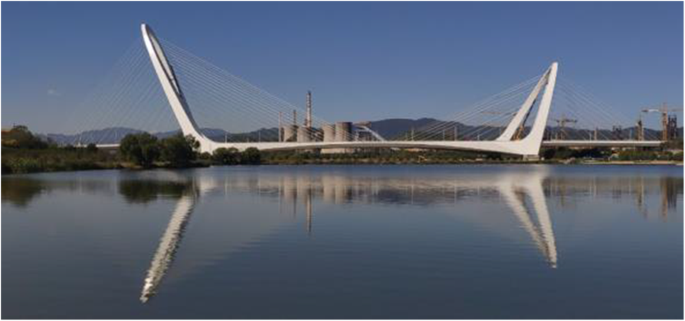The image depicts an elaborate, modern-design bridge spanning across a calm body of water, possibly a lake or river, with its reflection creating a symmetrical and ethereal effect. The bridge features a sleek, arched white frame with two large, eye-of-the-needle shaped arches on either side, from which cables descend at an angle, giving it the appearance of a loom used in fabric making or resembling the shape of a shoe. This engineering marvel is the focal point of the scene. In the background, there is a large power plant, potentially a nuclear facility or steel mill, with no smoke visible from its towers, suggesting it might be inactive. Surrounding the bridge are lush vegetation and greenery along the shoreline, accompanied by the distant silhouette of a small mountain. The clear blue sky and bright sunlight enhance the clarity and detail of this panoramic view.